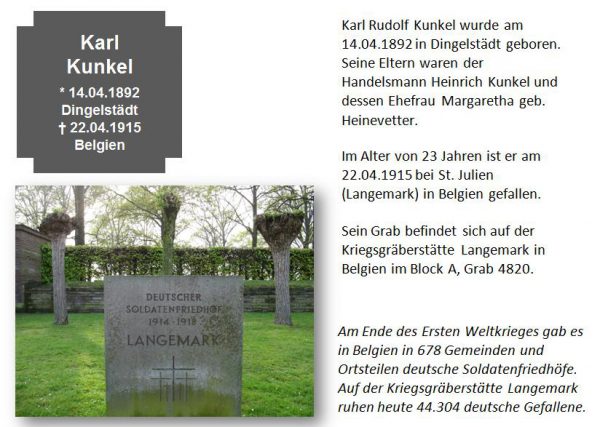This detailed caption describes a visually rich and intricate collage that depicts a solemn and poignant scene of remembrance:

The image is a collage blending a photograph and various text elements, suggestive of an obituary. In the lower left-hand corner lies a photograph of a tombstone situated in a green grass cemetery, surrounded by shrubbery and trees. The tombstone prominently bears the inscription "Deutscher Soldatenfriedhof" and "1914-1918 Langemark," along with the name "Deutscher" and a lengthy surname ending in "S". An illustration of several crosses adorns the tombstone.

In the upper left quadrant of the collage, the name "Karl Kunkel" appears with the dates "14.04.1892 Diengels" and "22.04.1915 Belgium", signifying birth and death dates respectively. 

The right half of the collage features text in German. It includes the name "Karl Rudolf Kunkel, Wörter Emmet" and seemingly outlines the life, death, surviving family members, and possibly details about the funeral of Karl Kunkel. The text transitions from regular script to italics towards the bottom.

The background of the scene extends to reveal additional cemetery details: three pillars filled with flowers in front of a bushy hedge, and trees in the distance, contributing to the tranquil and respectful environment.